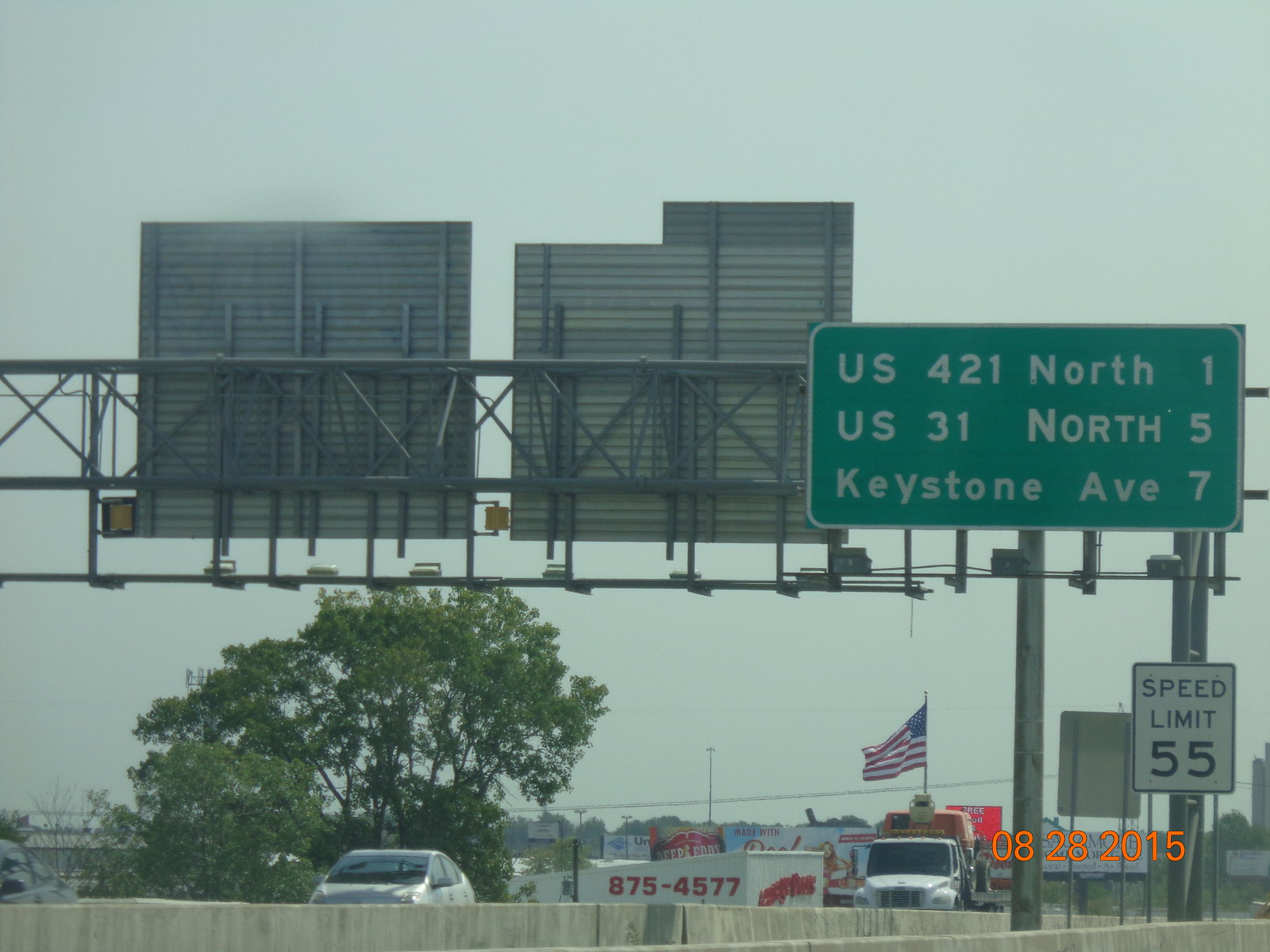A photograph captured on a freeway dated 08-28-2015, as indicated by the watermark in the bottom right corner. Prominently displayed at the top are several traffic signs mounted on metal poles. The signs on the left and center are viewed from their reverse sides, revealing only their metal framework. The sign on the right reads "US-421," followed by directional indicators for "North 1," "US-31," "North 5," and "Keystone Avenue 7." Beneath these, a white speed limit sign indicates a maximum speed of 55 mph. The image captures a typical roadside scene with essential navigational information and speed regulations for drivers.